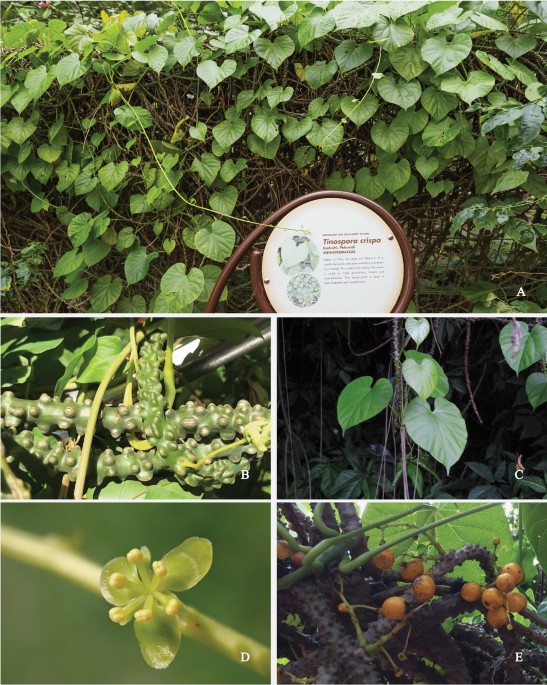The image showcases a collage of five photographs, each depicting various stages and features of a plant. The largest photo at the top reveals a lush bush with heart-shaped green leaves, accompanied by a white sign featuring some unreadable text. Directly below this, the bottom row is composed of four smaller photos. The bottom right photo highlights branches laden with orange, circular berries. To its left, a photo of a stem dotted with peculiar-looking bumps, possibly berries before they fully bloomed, adds an odd texture. The adjacent left image presents a mix of green leaves and a singular green bud. Throughout the collage, the progression from leafy vines to budding and fruiting stages encapsulates the varied life cycles of the plant.